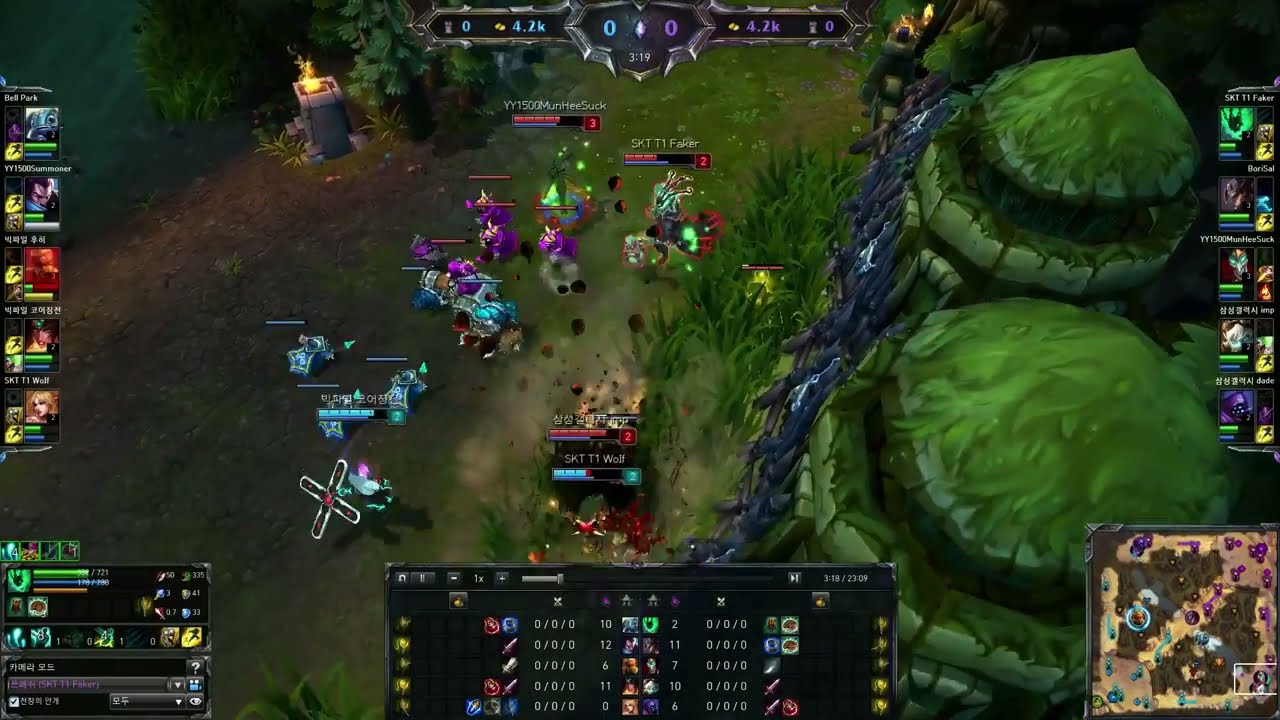This image is a detailed screenshot from the computer game League of Legends. The scene primarily showcases a marshy, jungle-like outdoor environment filled with elements such as grass, lily pads, water, and various green plants, which create a lush landscape. Dominating the center of the screen is a character named SKT T1 Faker, identifiable by a small health bar and an outfit featuring a combination of green and pink. The background includes both dark and earthy tones, with spruce trees and other foliage scattered throughout. 

On the right side of the image, there is a vertical column of icons representing different characters, each accompanied by blue and green health bars. The lower-right corner displays a detailed map overview, featuring icons representing multiple characters positioned around the terrain, illustrated with purple and blue highlights. Additionally, user interface elements such as scores, numerical data, and various icons are spread across the screen. Notably, there are blocks in the lower corners, with the lower-left corner containing bars indicating health or resources, and the lower-middle section featuring more numbers and icons in a black box.